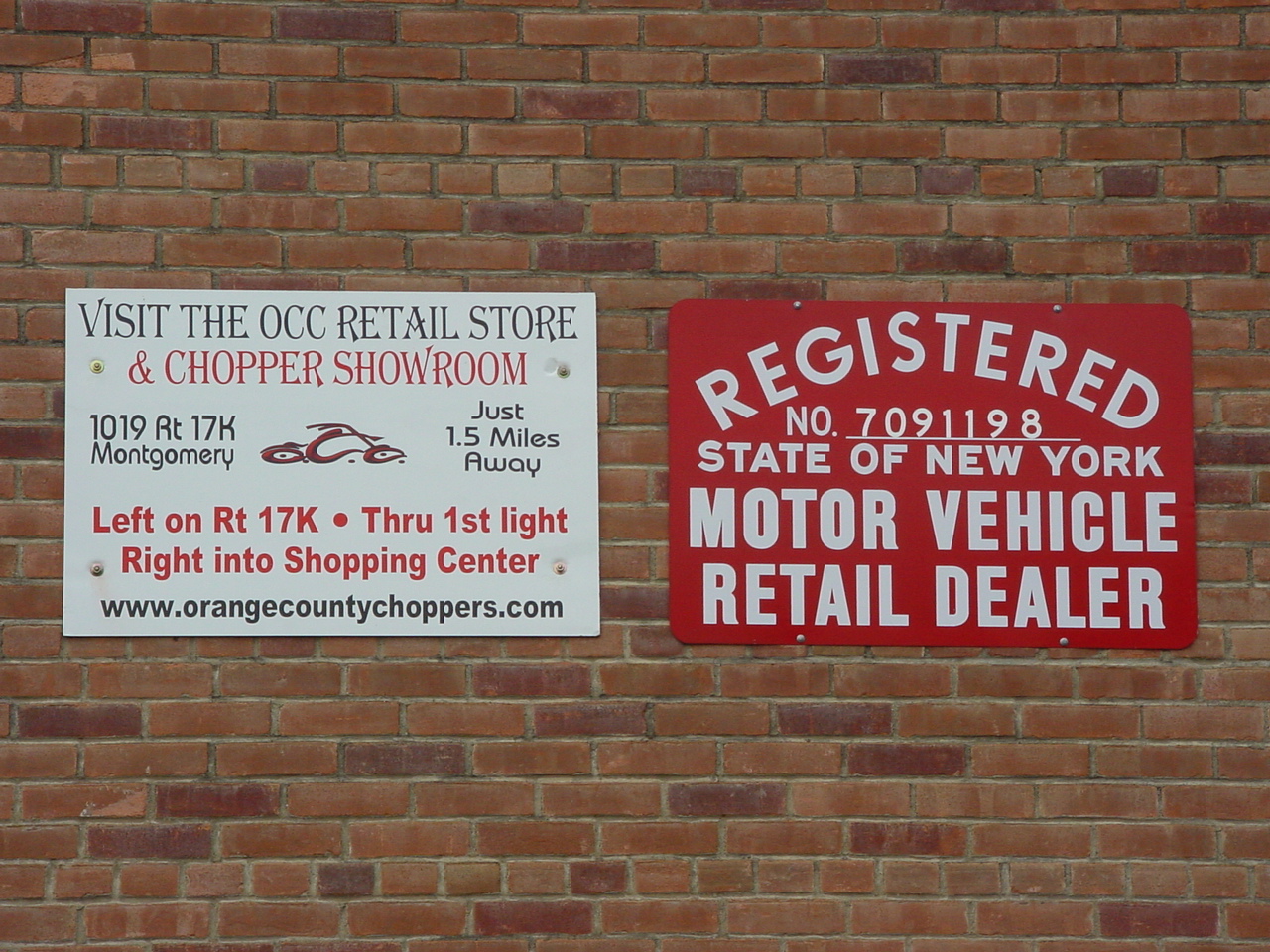The photograph depicts a traditional red brick wall featuring two distinct rectangular signs. The sign on the left has a white background and is adorned with a mix of black and red text, along with a logo of a red motorcycle. The top of the sign reads "Visit the OCC Retail Store" in black capital letters, followed by "and Chopper Showroom" in red text. Below this, the black text states "1019 RT 17K Montgomery" with a red motorcycle logo to its left, and "Just 1.5 miles away" in black to its right. Further down, in red text, it directs "Left on RT 17K through First Light, right into Shopping Center." The bottom of the sign features the website "www.orangecountychoppers.com" in black. This sign is secured with four brass screws, two on each side. To the right of this sign is another sign with a red background and white text. It displays in an arc "Registered," followed by the underlined number "709-1198." Below this, it reads "State of New York Motor Vehicle Retail Dealer" in stacked lines. This red sign is fastened to the wall with four silver screws, two at the top and two at the bottom. Both signs promote a motorcycle dealership and retail store affiliated with Orange County Choppers.